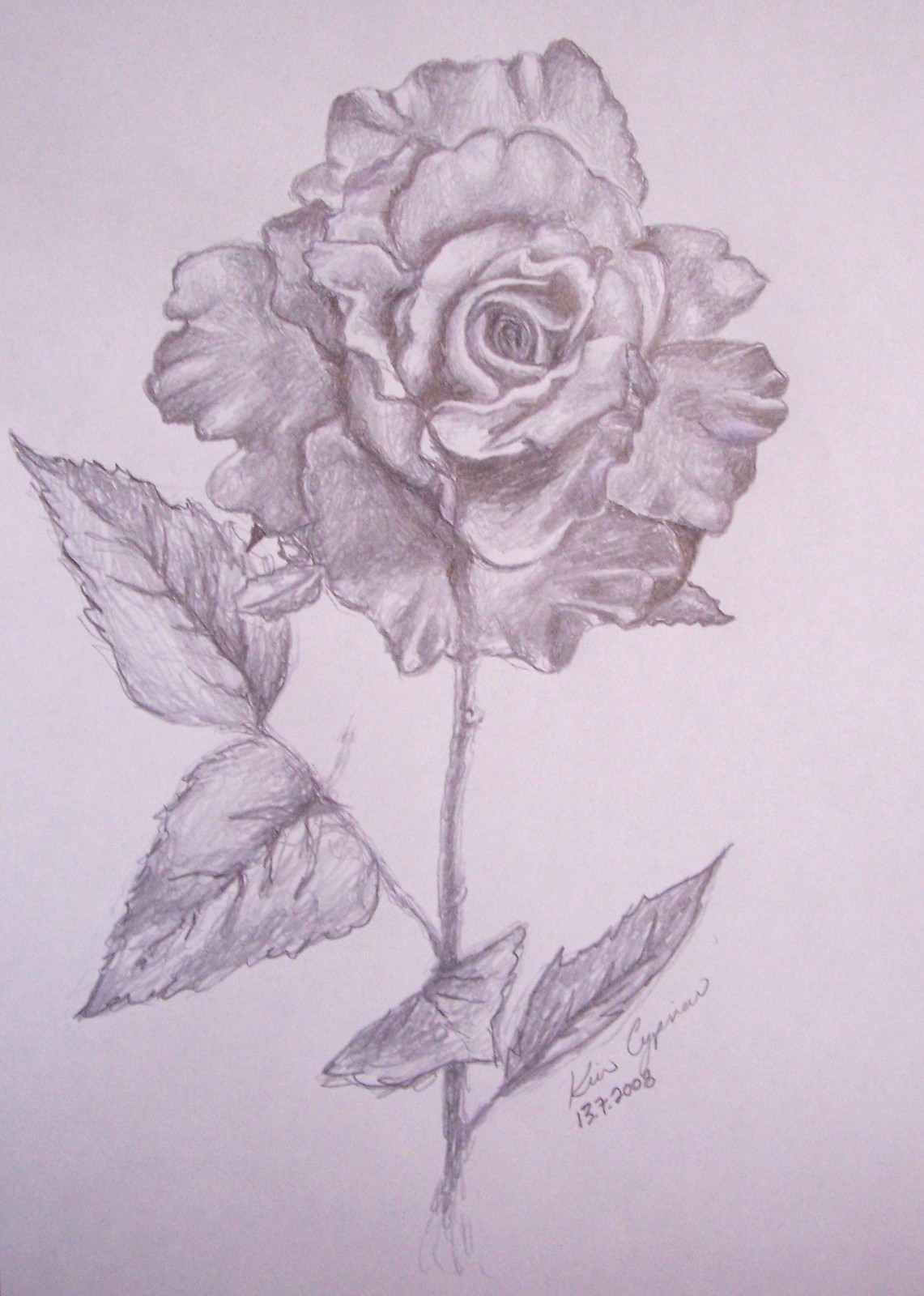The image is a vertically rectangular pencil sketch set against a faint lavender background. Central to the composition is a single rose with its stem reaching upward, originating from the bottom of the frame and stopping at the center. Midway up the stem, two leaves extend to the right. Progressing further up the stem, there is an additional sprout featuring two larger leaves; one leaf extends downward to the left, and the other extends upward to the left. Crowning the stem is a large, detailed, and fully bloomed rose that serves as the focal point of this delicate and intricate artwork.